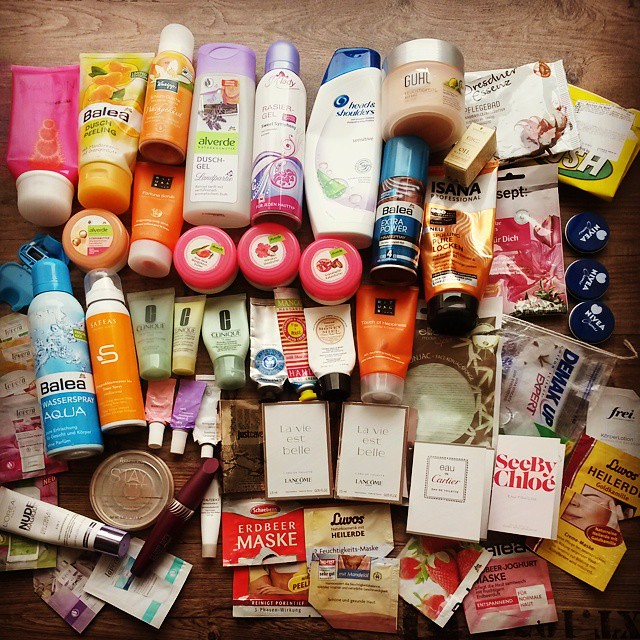This top-down photograph showcases an extensive collection of hair and personal beauty products, typically found in a bathroom, arranged on a medium to light-toned wooden surface with noticeable texture. The wooden background is prominently visible at the top of the image and peeks through in several places among the clustered products.

The arrangement starts relatively organized at the top and becomes more cluttered toward the bottom. In the top left corner, there is a bright pink squeeze bottle with a white cap. To its right is a green, white, and orange bottle labeled "Balia." Adjacent to this is a smaller orange aerosol or travel can adorned with a white flower. Continuing to the right, a purple-capped body wash bottle is visible.

The central and lower portions of the image feature a variety of items, including different shampoos and numerous small, travel-sized face washes. The bottom left section contains various makeup products, such as a blush tin and a mascara wand. On the right side, several lotions can be seen, including a couple of Nivea tins. The overall shape of the arrangement is approximately rectangular, encompassing a diverse array of beauty essentials.